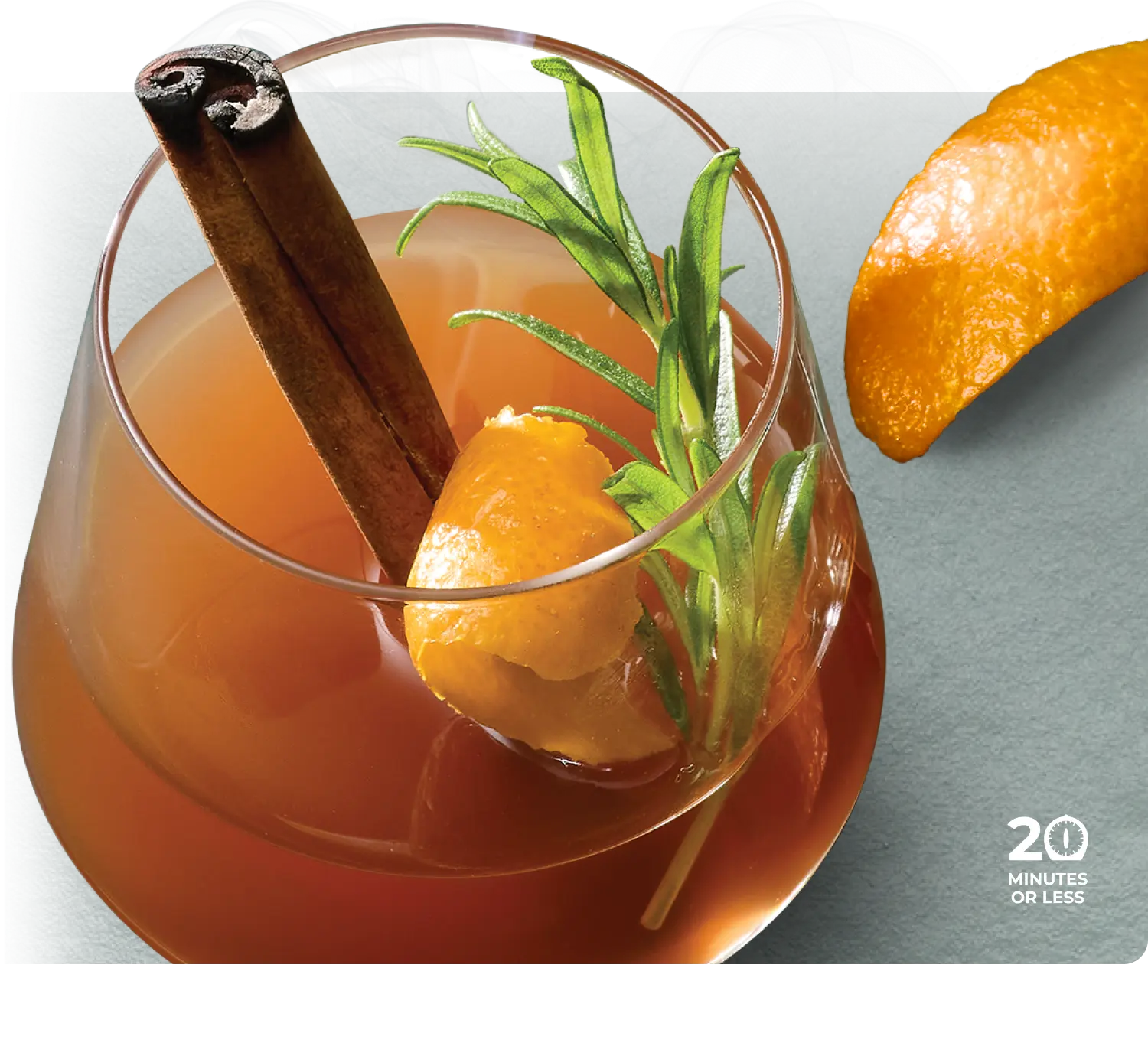The image features a close-up, top-down view of a sophisticated orange-hued cocktail, possibly intended for an advertisement or a cocktail recipe book. The drink is presented in a small glass on a gray, stone-like surface. Dominating the center of the image, the cocktail's intricate details include an orange rind both inside and outside the glass, a cinnamon stick, a sprig of green mint, and a potential hint of rosemary, suggesting a blend of flavors. The liquid within the glass has a rich, amber to brown coloration, hinting at a cider or juice base. In the bottom right corner, white text reads "20 minutes or less" with the "0" stylized as a timer, indicating the drink can be prepared within this timeframe. The overall background is gray, with a secondary note of an orange rind placed next to the glass, enhancing the drink's presentation and appeal.